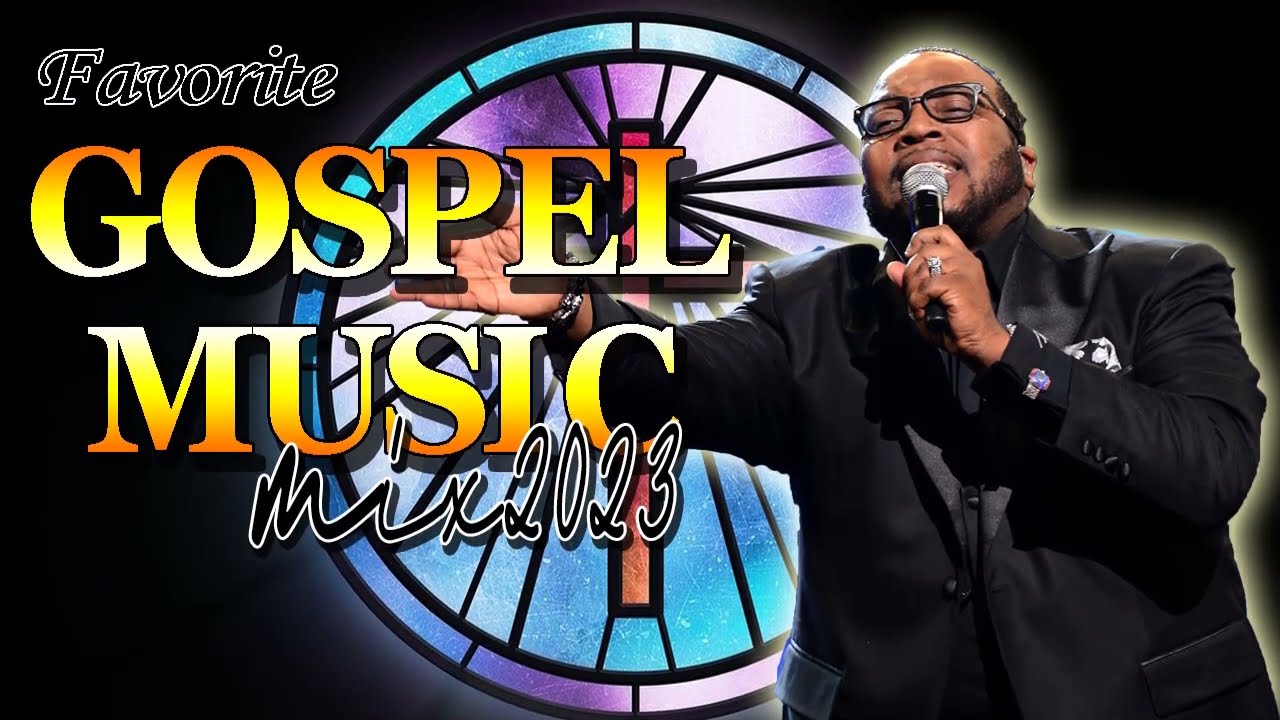The image, designed in a landscape format with a black rectangular background, appears to be an advertisement or album cover. Dominating the center of the image is a circular stained glass motif, primarily featuring blue and purple hues, with a prominent red cross at its heart. Overlaying this central design on the right is a well-dressed man of African descent in a shiny black suit, black shirt, and tie. He is wearing glasses and holding a microphone in his left hand, appearing to sing or preach, with his right arm outstretched. The text, positioned on the left-hand side, reads "Favorite Gospel Music Mix 2023." "Favorite" is at the top in black text with a white outline, while "Gospel Music" is displayed in a larger, blocky font with a gradient from orange to yellow to white. Beneath, "Mix 2023" is written in a curvy black font with a white outline.